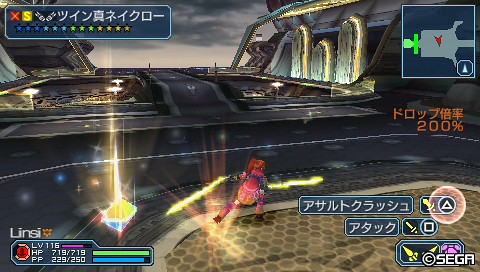This color screenshot captures a detailed scene from a Japanese role-playing video game developed by SEGA. Central to the image is a female protagonist with long red hair tied in a ponytail, dressed in a striking red dress with pink and orange hues. She is captured mid-action, seemingly lunging to the right while holding two lightsaber-like weapons glowing with yellow streaks of light. Her boots are a mix of red, orange, purple, and brown at the bottom.

The setting appears to be a large man-made platform, reminiscent of a spaceship or aircraft carrier, colored in dark gray and black. This platform is lined with various structures in green, yellow, and olive green, interspersed with sections that resemble open engine areas emitting green and yellow light.

In the interface, the protagonist's stats are displayed on the left with the name "L-I-N-S-I," indicating a level 116 character with full health (HP 719/719) represented by a green bar, and partial energy points (PP 229/250) shown with a blue bar. A glowing golden object with blue accents lies on the ground nearby, hinting at a possible collectible or interactive element.

Additional gameplay information is scattered around the screen, including Japanese text and a 200% indicator in orange. The top of the screen features a legend with white Japanese characters, a red 'X,' a yellow 'S,' and a row of stars in various colors—three dark blue, three cyan, three green, and four gold. A minimap occupies the top right corner, and nearby, several rectangles with Japanese text and icons such as a yellow sword inside a blue rectangle and another sword next to a white square can be seen. A spear icon and a small symbol resembling purple armor are also part of the UI elements.

Finally, the bottom right corner displays "copyright SEGA" in white, confirming the game's publisher and adding a finishing touch to this vibrant and intricate scene.